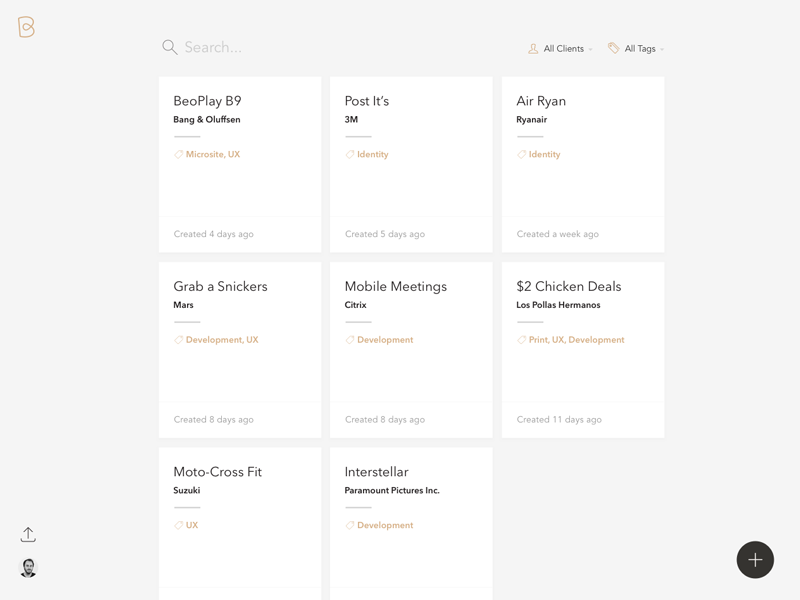This image is a detailed screenshot featuring a project management interface of an unnamed platform. At the top of the screen, several filters are visible: "Search," "All Clients," and "All Tags." Below these filters are a series of list items, each mentioning various projects along with their details such as title, client, category, and the date of creation. 

The listed projects are as follows:
1. **Beoplay B9** for Bang & Olufsen, categorized under "Microsite UX," created 4 days ago.
2. **Post-its 3M** for Identity branding, created 5 days ago.
3. **Air Ryan** for Ryan Air, categorized under "Identity," created a week ago.
4. **Grab a Snickers** for Mars, under "Development, UX," created 8 days ago.
5. **Mobile Meetings** for Citrix, under "Development," created 8 days ago.
6. **$2 Chicken Deals** for Los Pollos Hermanos, categorized under "Print, UX, Development," created 11 days ago.
7. **Motocross Fit** for Suzuki, under "UX."
8. **Interstellar** for Paramount Pictures Incorporated, categorized under "Development."

In the bottom left corner, there is an upward-pointing arrow next to a small, circular black-and-white photo of a man. The bottom right corner features a black circle containing a white plus sign in its center.

The image is devoid of animals, birds, plants, flowers, trees, automobiles, bicycles, airplanes, and boats.